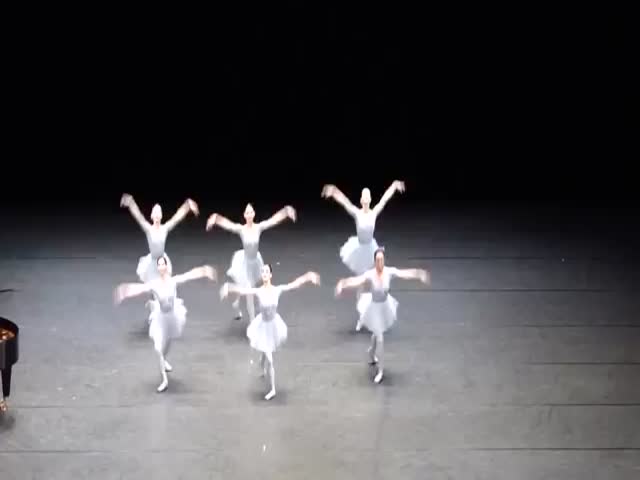The photograph captures a ballet performance featuring six Caucasian ballerinas dressed in identical white leotards, skirts, tights, and shoes, all with their hair pulled back. They are positioned on a dark gray or black stage floor, and the background is entirely black, likely due to stage lighting emphasizing only the dancers. The picture appears to be taken from a distance, possibly from an audience balcony, resulting in a slightly blurred focus. The dancers are all standing with their left foot forward and pointed to the side, while the right foot is pointed back, touching the floor. Their arms are raised in a bird-like motion, extending to the sides, creating a unified and graceful formation. On the very left edge of the image, the blurry outline of what appears to be a piano is visible. The spotlight on the dancers contrasts sharply with the dark surroundings, highlighting the synchronicity and elegance of the ballet performance.